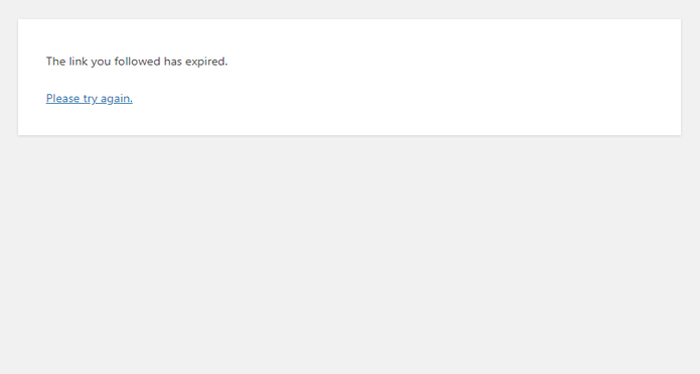The image features a light gray rectangular background that is longer in width than in height. Positioned at the top of this light gray rectangle is a smaller white rectangle, which occupies about one-third of the area of the larger rectangle. The white rectangle is also longer in width than in height. Within the white rectangle, the text "The link you followed has expired." is centrally aligned and written in black font. Directly below this message, the phrase "Please try again." is displayed in blue, underlined text. The overall color palette of the image consists of light gray, white, black, and blue. The composition is minimalistic, containing no additional elements or decorations.